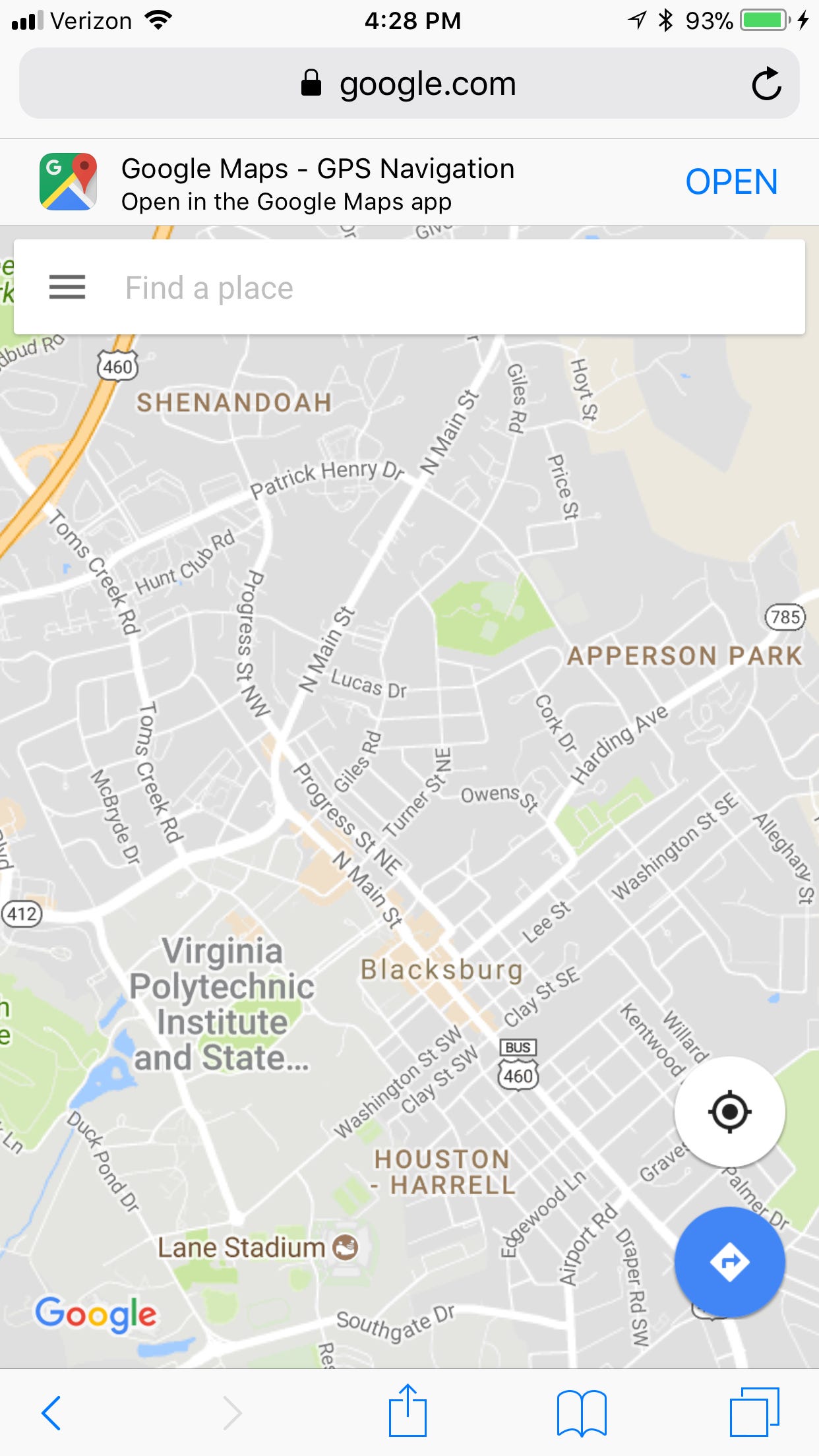The screenshot captures a detailed view of a cell phone screen at precisely 4:28 PM. In the top right corner, the battery icon indicates a robust 93% charge, and the Bluetooth feature is activated. The top left corner shows connectivity information, with the Verizon network and Wi-Fi signal icons both visible. 

Beneath these icons is a search bar from Google.com, complemented by a refresh button on its right side. Directly below the search bar sits a banner advertisement for Google Maps GPS navigation, which includes an "Open in the Google Maps app" prompt accompanied by an "Open" button on its right.

Further down, a "Find a place" search field is present, marked with three vertical lines signifying a menu option. The main portion of the screen is occupied by a map, likely depicting an area in Texas, given the visible "Houston" marker and directional arrow pointing towards it.

Finally, the bottom section of the screen displays a navigation bar with various icons: a back arrow, a forward arrow, an upload button, an image of a book, and a couple of square icons, likely indicating additional functionality or apps.